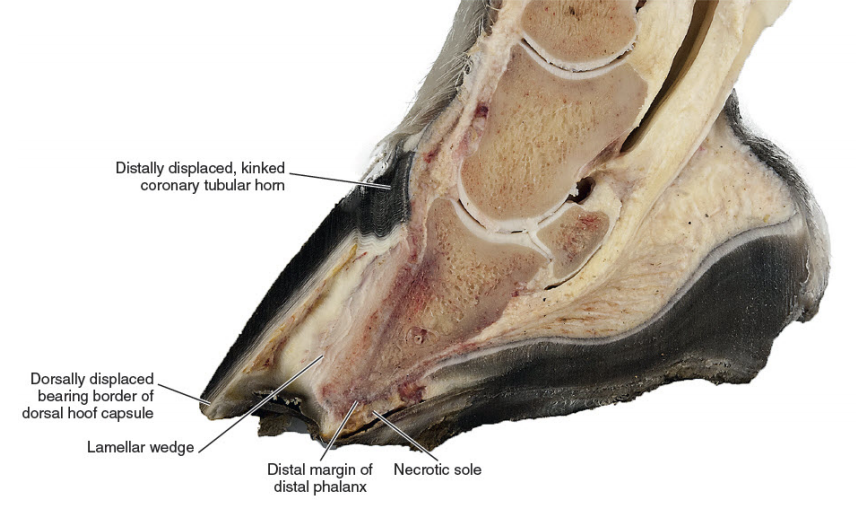The image depicts a detailed cutaway view of an ungulate's hoof, most likely from a horse or deer. The hoof has been longitudinally sliced, exposing various internal structures and components. The exterior shows the characteristic hairline at the top, transitioning down to the keratinous part of the hoof. Inside the cutaway, several labeled parts are visible: the "distally displaced kinked coronary tubular horn," the "dorsally displaced bearing border of the dorsal hoof capsule," the "lamellar wedge," the "distal margin of distal phalanx," and the "necrotic sole." The hoof appears to be dissected from a cadaver, and though it's a clinical image with no blood, the black, white, and flesh-colored tissues give a somewhat grotesque impression. The labels provide precise identification of each anatomical component, useful for educational purposes.